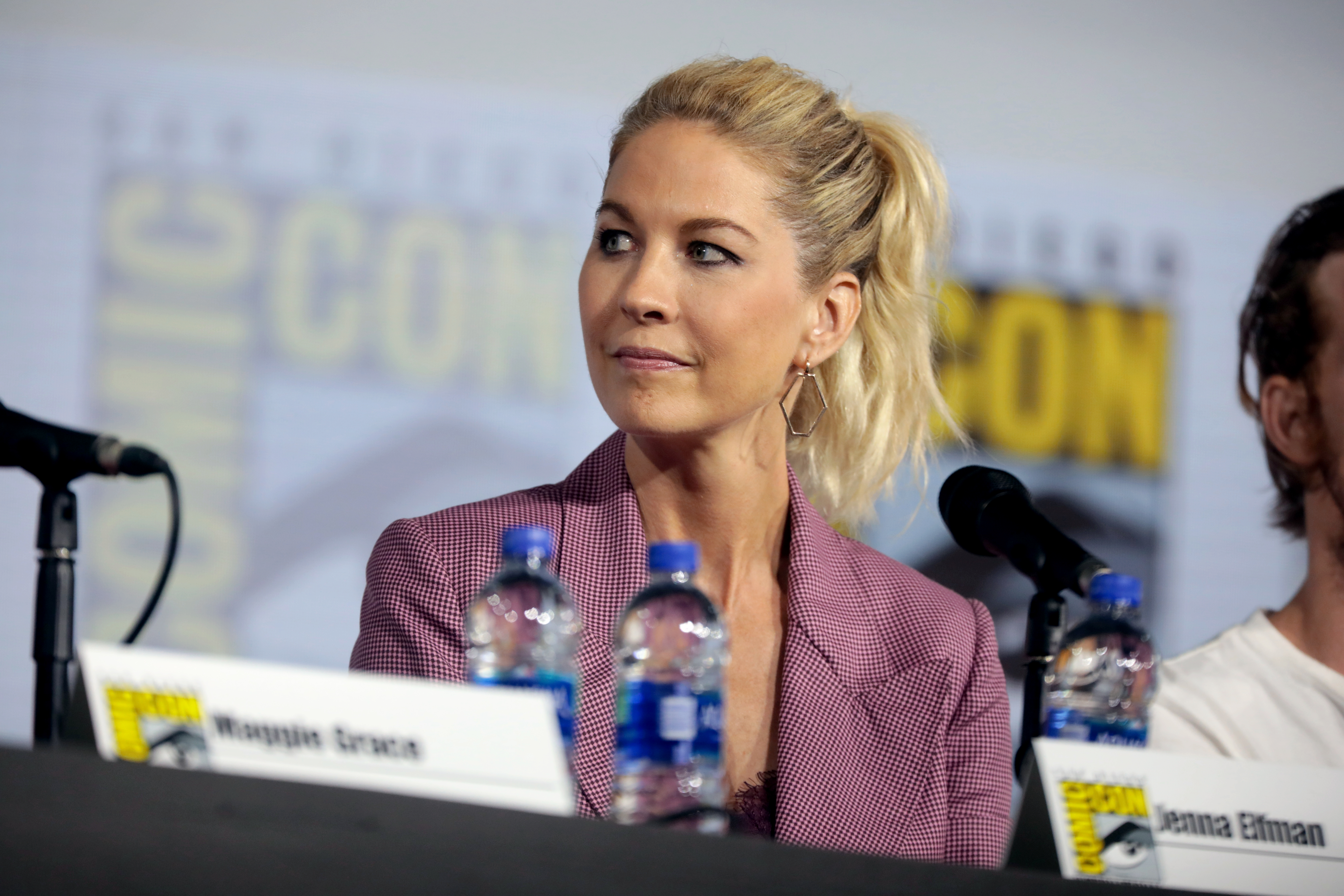In this detailed close-up photograph, we see an elderly blonde woman named Jenna Eifman, as indicated by her white name tag with her name in black text. She is seated in front of a microphone at what appears to be a convention or event, possibly Comic Con, with the event name in yellow text on her name tag. The word "Comic" is uniquely oriented 90 degrees counterclockwise, forming an 'L' shape with the word "Con" placed at the top. Jenna has her hair styled in a high ponytail and is wearing a dull raspberry-colored suit jacket over a blouse. Her makeup includes notable mascara and eyeshadow, and she accessorizes with hexagon-shaped gold earrings in her right ear. In front of her on the table are three water bottles. To Jenna’s right, a man with dark brown hair, sideburns, and a white t-shirt is partially visible, though his face is cut off in the image. They are indoors, seated at a table, with a backdrop behind them, suggesting a speaking event or panel discussion. The colors in the image include dark pink, blonde, brown, black, blue, royal blue, yellow, and off-white.